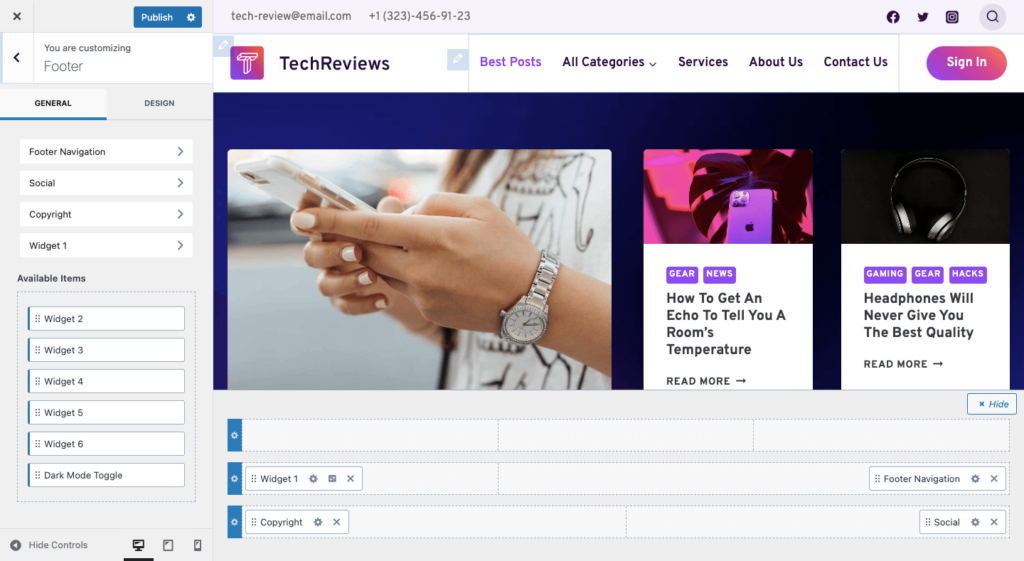Screenshot of a web page customization interface. On the left-hand side, there's a vertical gray box with a small blue "Publish" button at the top. Below it, white boxes indicate the user is customizing the footer section, with two tabs underneath: "General" and "Design." The "General" tab is underlined in blue, indicating it is currently open. 

Four menu options are displayed beneath: "Footer Navigation," "Social," "Copyright," and "Widget 1." Additional items listed below include "Widget 2," "Widget 3," "Widget 4," "Widget 5," "Widget 6," and "Dark Mode Toggle." At the bottom of the screen, there's an option to "Hide Controls" and three icons representing desktop, tablet, and mobile phone views.

On the right-hand side, the top bar showcases an email (techreview.email.com) and a phone number (+1 323-456-9123). Social media logos for Facebook, Twitter, and Instagram appear below. Further down, a white bar states "Tech Reviews" followed by a menu with options: "Best Posts," "All Categories," "Services," "About Us," "Contact Us," and a purplish orange "Sign In" button. 

The lower section features a prominent purple bar with an image of a woman's hands holding a phone. Adjacent to this are two images, one of a mobile phone and the other of headphones.